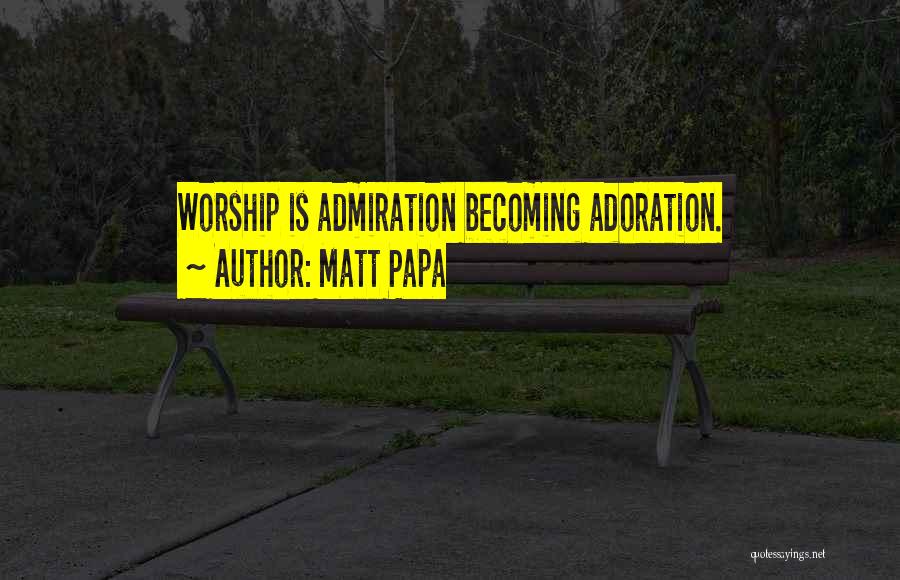A wooden park bench with light brown-grayish color and half-circle metal legs is positioned on a gray sidewalk. The bench is facing a field of vibrant green grass, which transitions into a lush forest background. The trees directly behind the bench are bare, with no leaves contrasting the fully leafed, healthy green trees further back. In the image, a quote is overlaid on yellow rectangles with black text that reads, "Worship is admiration becoming adoration." The author of the quote is Matt Papa, indicated below the text, followed by a squiggly line. At the bottom right corner of the image, in white text, it reads "quotesayings.net". The overall setting is serene and natural, with noticeable contrasts in foliage and a subtle depth created by the foreground and background elements. The image has a dark tone and slightly blurry, adding to its contemplative atmosphere.